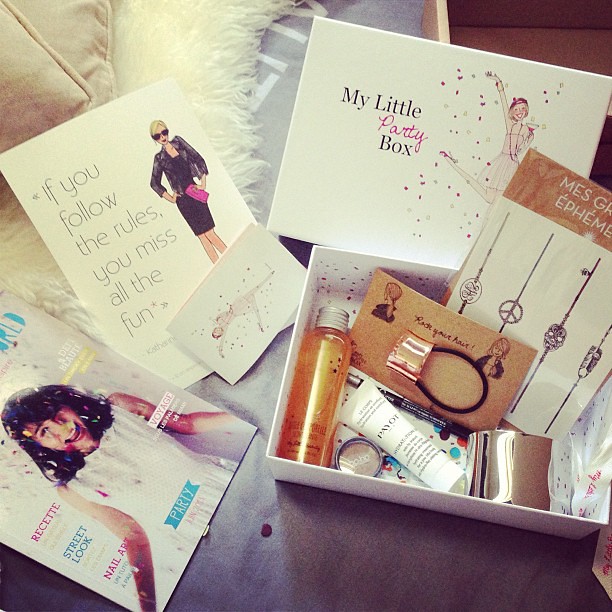The image depicts a collection of beauty and fashion items arranged around a white box labeled "My Little Party Box." The box’s lid, placed behind it, features a hand-drawn image of a woman celebrating with a martini glass, confetti falling around her, and the word "party" prominently in pink. The contents of the box, spread out across a table, include various beauty products such as a bottle of liquid, a tube of cream, and pieces of jewelry, likely bracelets. 

To the left of the box, several papers and postcards are visible. One postcard shows an illustration of a woman in a black dress holding a pink bag, accompanied by the caption, "If you follow the rules, you miss all the fun." Another paper features a smiling woman with confetti around her and colorful words like "Party," "Street Look," and "Nail Art." A magazine is partially visible on the left side, showing the cover image of a woman with dark hair in a white dress. The scene appears to be set on a couch adorned with pillows and faux fur, suggesting an intimate, cozy setting for party preparations or a celebratory event, possibly for a girl's night or birthday.

Overall, the detailed arrangement and specific thematic elements indicate that the contents of "My Little Party Box" are intended for party preparation, offering items such as makeup, hair accessories, and fun, decorative postcards to enhance the celebratory experience.